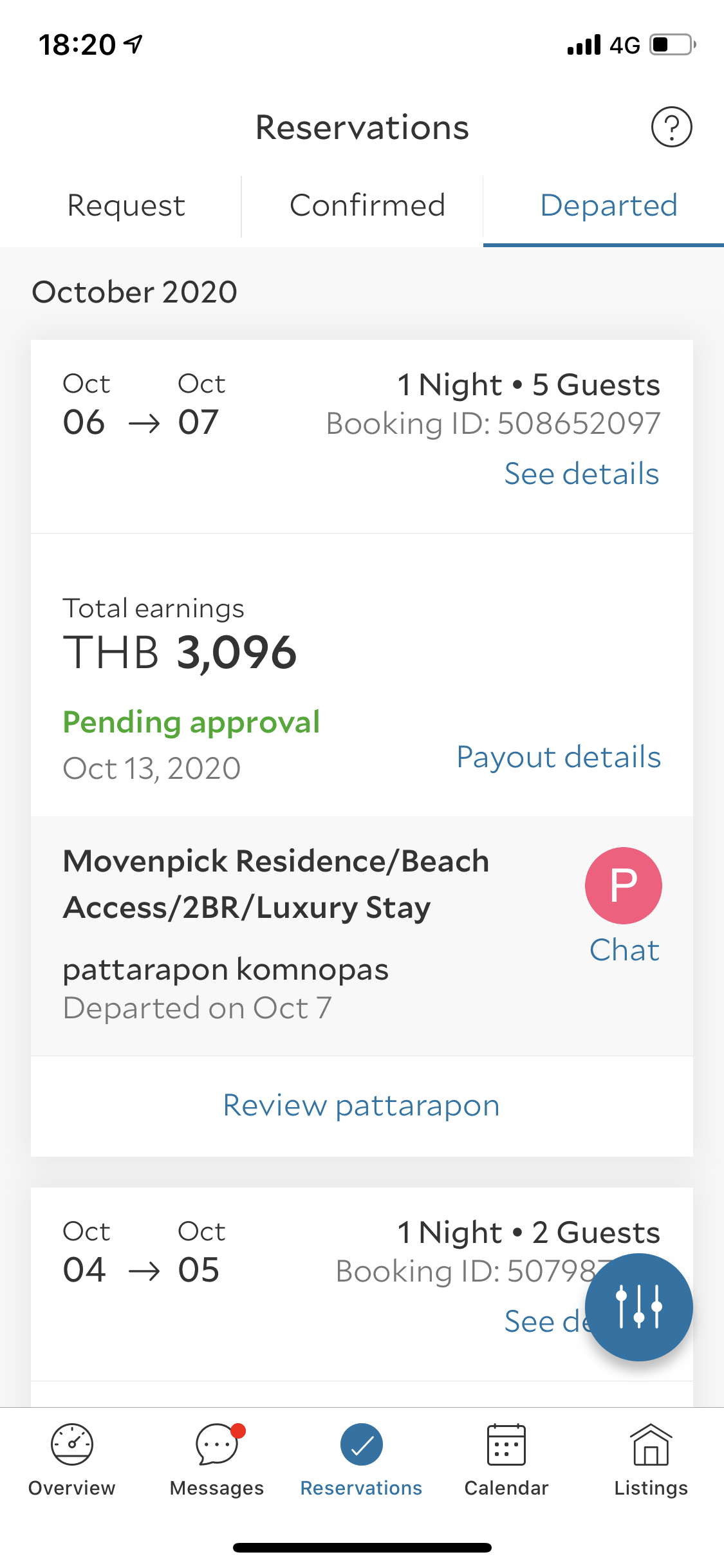The screenshot showcases a reservation management page for a property listing. At the top, the page is titled "Reservations," featuring three columns labeled "Call Request," "Confirmed," and "Departed." The details for a specific booking are highlighted: the reservation spans from October 06 to October 07, 2020, for one night accommodating five guests. The booking ID is provided, along with total earnings of THB 3,096. Additionally, a note indicates that approval is pending, with payout details set for October 13, 2020.

Further down, the reservation details include the property name "Morvan Peak Residence Beach," described as offering "luxury stay." A guest named Pata Rapan Kamnoupas departed on October 07. There is also an option to review Pata Rapan Kamnoupas.

Below that, another booking is detailed for October 04 to October 05, 2020, for one night and two guests, with a separate booking ID. At the bottom of the page, navigation options are listed: "Overview," "Messages," "Reservations," "Calendar," and "Listings."